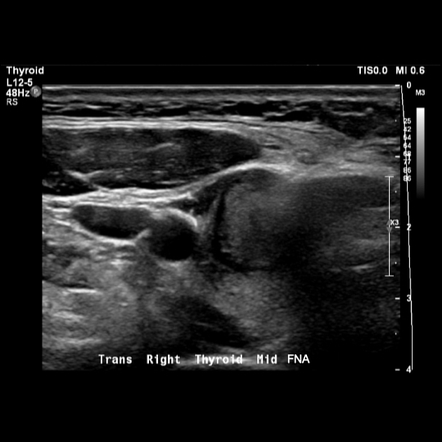The image is a black-and-white ultrasound of a thyroid. The ultrasound occupies the center of the image with varied white, black, and gray sections indicating different tissue densities. At the top left, a label reads "Thyroid, L12-5, 48 Hz, RS." To the top right, the text reads "TISO.0, MI0.6," followed by "0 M3." A bar or legend on the right side of the image transitions from white at the top to black at the bottom, with adjacent numbers ranging from 25 to 86, followed by 2, 3, and 4 in white. At the bottom of the image, the label "trans-right thyroid mid-FNA" is prominently displayed in white text. Overall, the image is characterized by its grayscale aesthetic and diagnostic details.